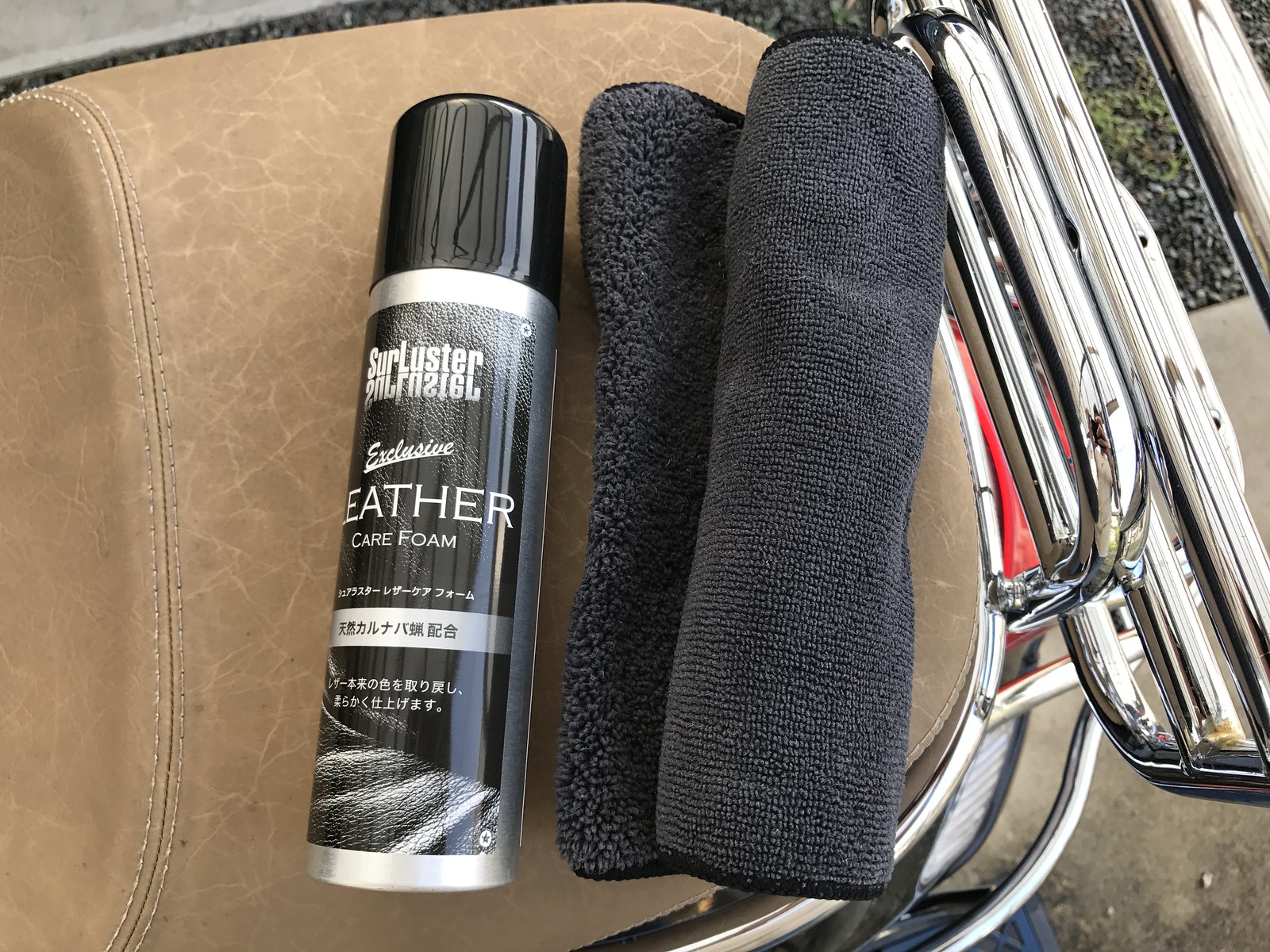The image depicts a detailed scene featuring a chair, possibly in a backyard setting, with various objects arranged on it. The chair is upholstered in crinkled and veined beige leather and has a shiny chrome and metal frame. Two cleaning cloths, one dark gray microfiber towel neatly wrapped and the other grayish in color, are placed on the chair. Next to these cloths, there is a silver spray can with a black cap. The can is labeled in English with "Sir Luster Exclusive Leather Care Foam" in white text, and it also features additional writing in possibly Chinese or Japanese. The chair is set amidst a tiled area with small rocks visible in the scene, suggesting an outdoor environment. Stainless steel pipes are seen in the background.